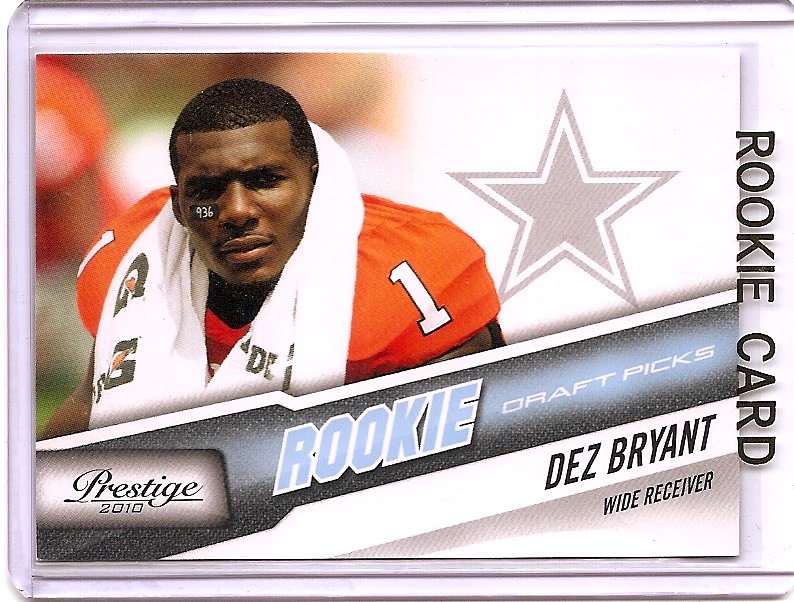The image is of a horizontally placed American football rookie trading card featuring Dez Bryant, the wide receiver. The card is encased in a clear plastic protector with "Rookie Card" written vertically in black along the right edge. On the card, "Rookie Draft Picks" is prominently displayed above, followed by the Dallas Cowboys star emblem in the upper right corner. Dez Bryant, in an orange college football uniform with the number one on the shoulders, is depicted on the left side. He has a white towel with a Gatorade logo around his neck, black paint under his left eye with the numbers 936 in white, and short black hair. The bottom part of the card features a blue and gray strip reading "Prestige 2010", and below this, in a coppery-colored banner, is written "Rookie". On a white line stripe below, it says "Des Bryant" and then "Wide Receiver" in a dark gray to white gradient.